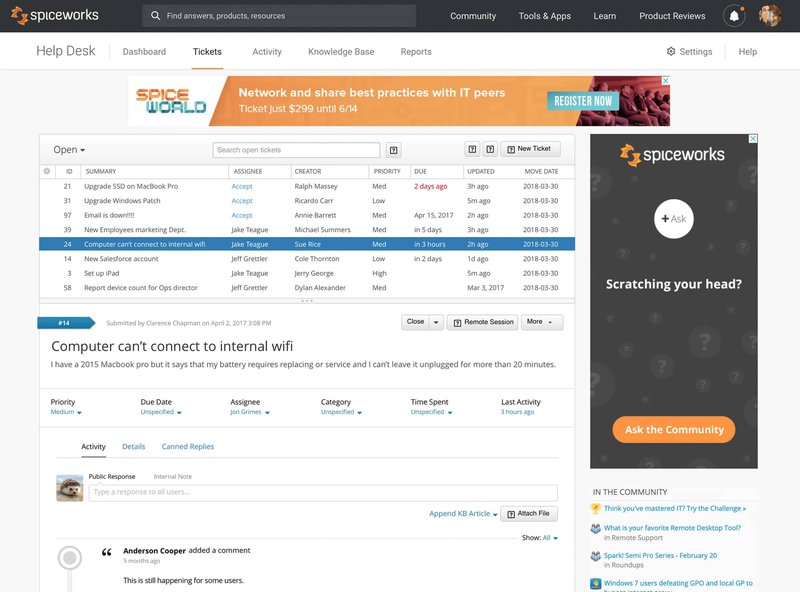The image displays a screenshot of a website with a clean, white background. At the top of the page, there is a black horizontal navigation bar. On the left side of this bar, the word "Spiceworks" is prominently featured in white text. Just below this bar, the gray text indicates our current location on the site: "Help Desk."

The navigation bar includes several tabs: "Dashboard," "Tickets" (which is underlined in orange to show it's the selected tab), "Activity," "Knowledge Base," and "Reports." Directly below these tabs, an orange bar spans the width of the page, displaying the word "Spiceworld" towards the left side.

The main content area features a window that lists several open help desk tickets. Ticket number 24 is highlighted with a blue background, making it stand out. Below this ticket number, a message in black text indicates the issue at hand: "Computer can't connect to internal wi-fi."